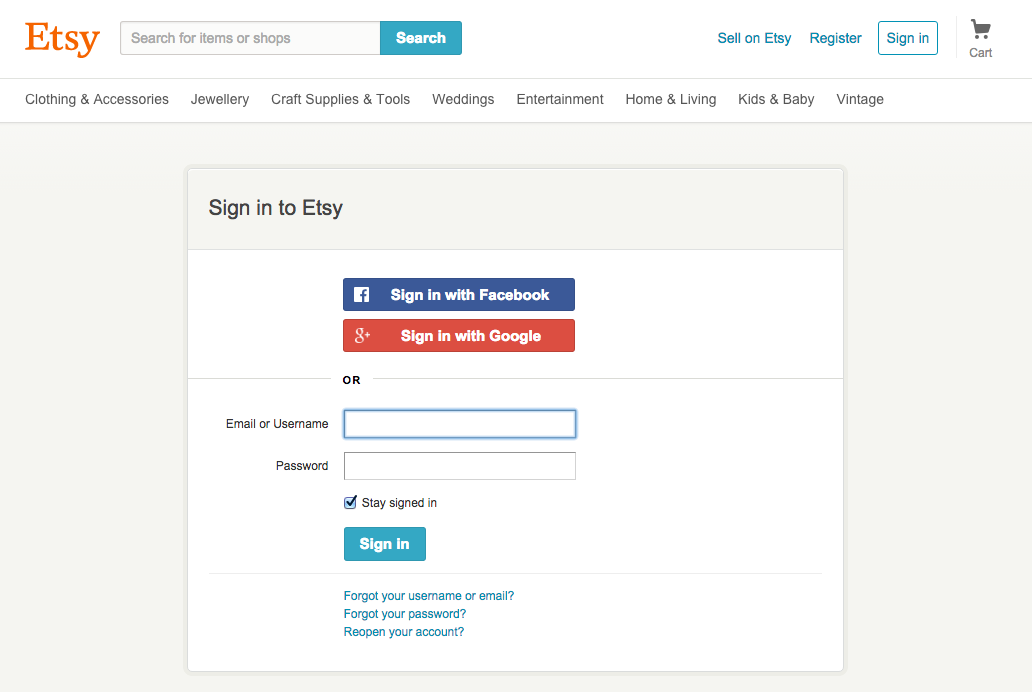The image appears to be a screenshot of the Etsy login page. The upper portion of the background is predominantly white, with the upper left corner highlighted in orange, featuring the Etsy logo with a capital 'E'. Adjacent to the logo, there is a light gray search bar with a 'Search' label on a white background on the right end.

To the right of the search bar, the navigation bar continues with a blue 'Sell on Etsy' link, followed by 'Register' and 'Sign in', all enclosed in a rectangular outline. Next to this is a gray vertical line, followed by a gray shopping cart icon with the word 'Cart' beneath it.

Below this primary section, a thin gray horizontal line traverses the width of the image, separating different navigational tabs for categories such as 'Clothing and Accessories', 'Jewelry', 'Craft Supplies and Tools', 'Weddings', 'Entertainment', 'Home and Living', and 'Kids and Babies'.

The main area of the image displays the login section. This area has a mostly white background with a gray header on top. The header contains the text 'Sign in to Etsy' in black. Below, there are two prominent buttons: a blue rectangle labeled 'Sign in with Facebook' and a red rectangle labeled 'Sign in with Google'.

Underneath these buttons, there is an input field for 'Email or username', followed by another field for 'Password'. Both fields are highlighted in blue on a white background. There's a checkable blue box with the text 'Stay signed in' next to it.

At the bottom of this section are additional links in blue text for users who have forgotten their password, username, or email, as well as options for reopening an account.